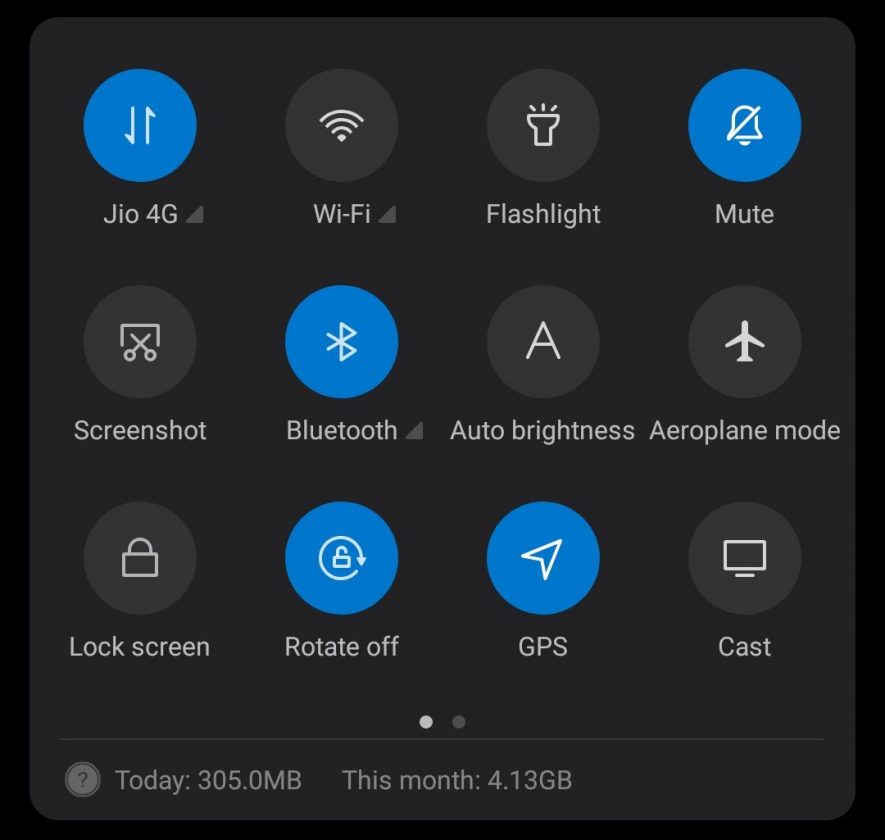The image depicts a smartphone screen showcasing a webpage with various toggle options for controlling different settings. The screen is organized with an array of icons, each representing a specific feature that can be enabled or disabled. 

At the top left, the first icon is "GIO4G," illustrated as a blue circle with upward and downward facing arrows, indicating that this setting is active. Next is the "Wi-Fi" icon, designed as a series of concentric curves resembling a signal strength indicator, which is currently turned off. The "Flashlight" icon, depicted with light rays emitting from a graphic of a flashlight, is also off.

The "Mute" setting features a bell with a diagonal slash through it, signifying that the bell is muted; this icon is blue, meaning it is activated. The "Screenshot" icon appears next and is turned off. Following that, the "Bluetooth" icon is highlighted in blue, signifying that the Bluetooth function is enabled.

"Auto Brightness" is represented by another icon, which is currently switched off. Adjacent to it, the "Airplane Mode" icon is also disabled. The "Lock Screen" function is turned off, as indicated by its icon. Similarly, the "Rotate Off" feature, represented by a lock with an arrow in a circular motion around it, is not active.

The "GPS" setting, which is also highlighted in blue, is turned on, while the "Cast" feature, displayed as an icon of a computer screen, is inactive. 

At the bottom of the screen, there's a textual display providing data usage statistics: today, the usage is 305.0 MB, whereas for the month, it is 4.13 GB. This detailed layout efficiently informs the user of the current status and usage of various smartphone settings.